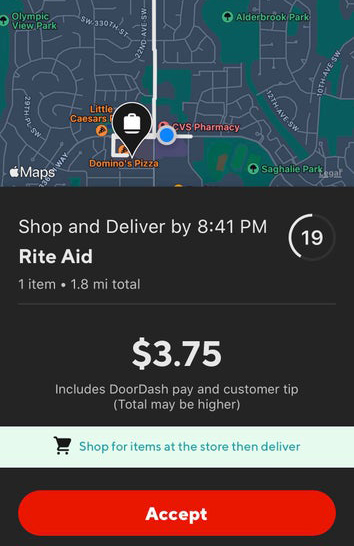The image is a mobile screenshot of a DoorDash information screen. The top third of the image displays a map, with an Apple Maps icon in the bottom left-hand corner. There is a prominent black location marker with a briefcase icon positioned over Domino's Pizza. Other locations marked on the map include Little Caesar's Pizza and CVS Pharmacy. A white line indicates the delivery route.

Beneath the map, there is a section with white text on a black background that states, "Shop and deliver by 8:41 PM, Rite Aid, one item, 1.8 miles total." On the right side of this text, there is a number "19" inside a half-circle. 

In the center of the image, large white text reads "$3.75," with a note underneath that this amount includes DoorDash Pay and Customer Tip, and the total may be higher. Below this is a light blue banner with a shopping cart icon and blue text that instructs, "Shop for items at the store then deliver."

At the bottom of the image, on a black background, there is a horizontal oval button filled in red, with white text in the center that reads "Accept."